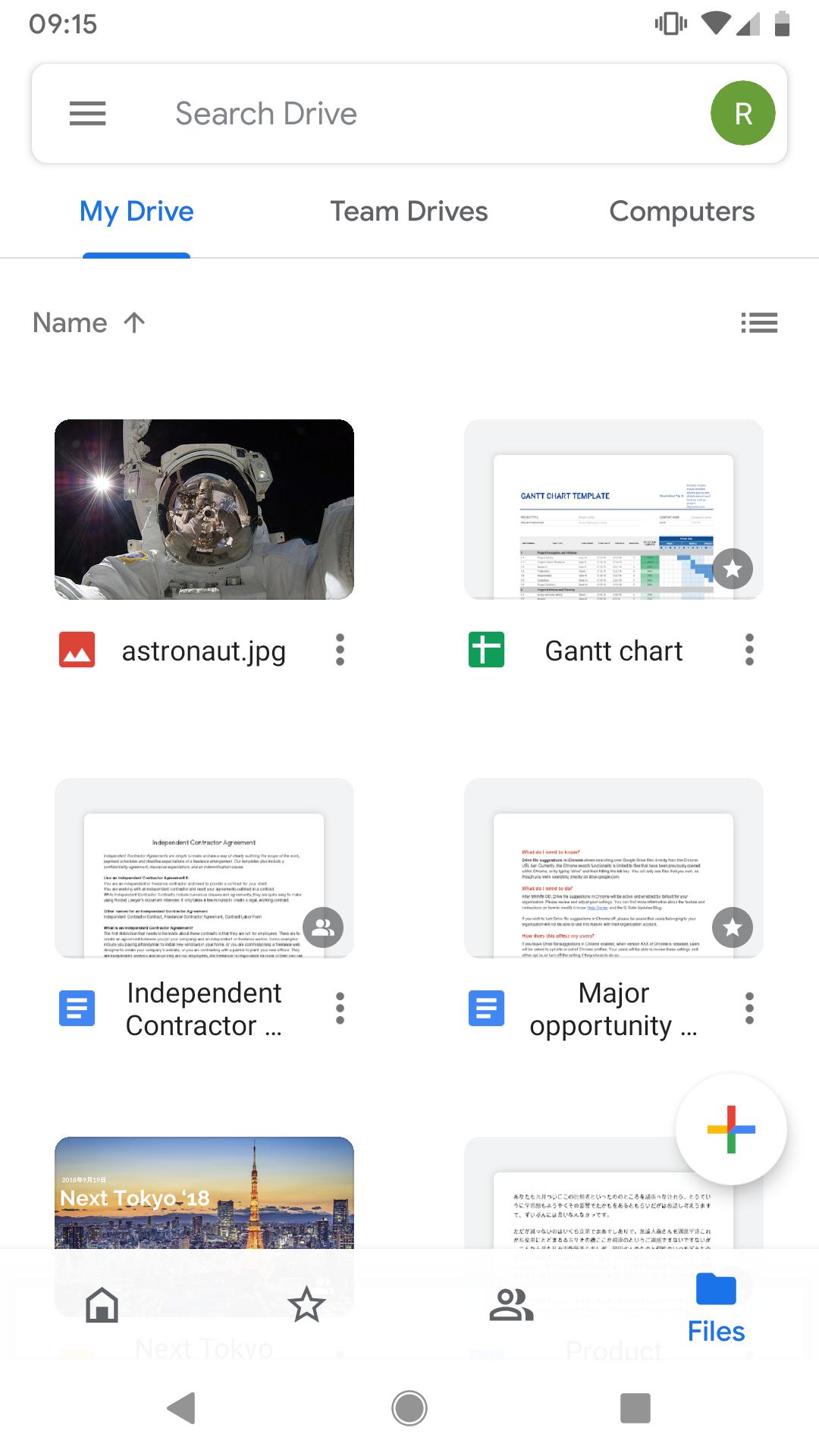This image is a screenshot taken from a cell phone in portrait mode, displaying a Google Drive interface against a white background. In the upper left-hand corner, the time is shown as 9:15, while the upper right-hand corner indicates a battery that is halfway charged. 

Beneath this, the screen shows a search bar labeled "Search Drive," with a three-line menu icon (commonly referred to as a hamburger menu) on the left and a green circular icon with the letter 'R' on the right. 

The next row consists of column headers: "My Drive," "Team Drives," and "Computers." "My Drive" is highlighted in blue, indicating it is selected. Following this, there's a row with sorting options: "Name," accompanied by an upward-pointing arrow, and a three-dot menu icon for additional settings on the right.

The main content area displays six items stored in Google Drive. The first item is an image file labeled "astronaut.JPG," featuring an astronaut in space with a celestial body, either the moon or sun, in the background. Adjacent to this is a file titled "GANTT chart," a spreadsheet partially visible in the image.

Below these, on the left, is a Google Doc named "Independent Contractor," specifically an "Independent Contractor Agreement." On the right is another Google Doc titled "Major Opportunity." 

The final row displays an image partially seen with the label "Next Tokyo 18," and to its right, a Google Doc appearing to contain Chinese characters.